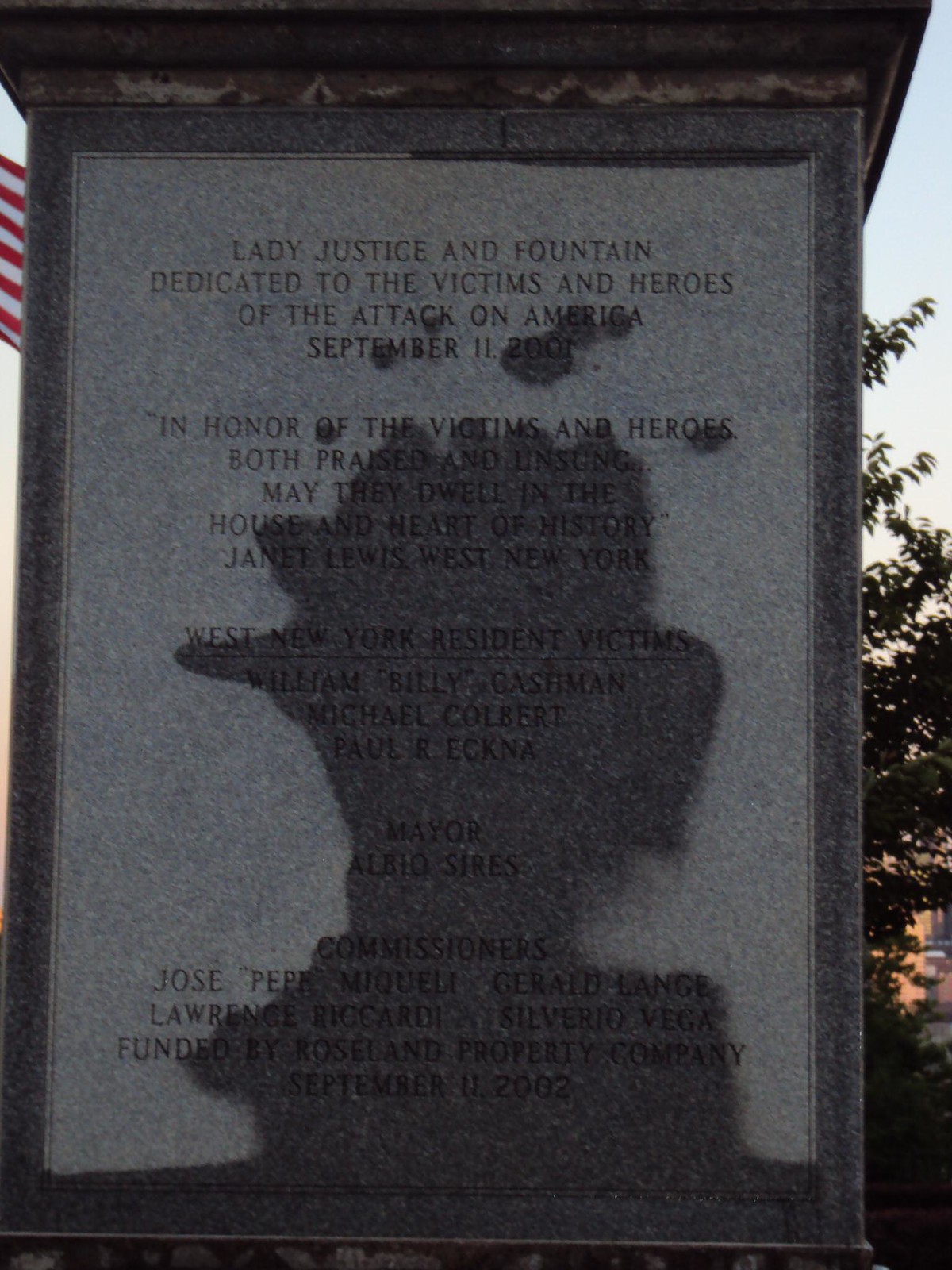The image captures a large, granite memorial dedicated to the victims and heroes of the September 11, 2001 attacks. The outer border of the stone monument is a dark gray, while the inner section is a lighter gray. A dark splotch, likely from water or the shadow of a nearby object, marks the center of the monument. In the background, part of the sky and a partially visible U.S. flag can be seen, as well as some trees. The engraved text on the lighter inner section of the memorial reads, "Lady Justice and Fountain, dedicated to the victims and heroes of the attack on America, September 11, 2001. In honor of the victims and heroes, both praised and unsung, may they dwell in the house and the heart of history." Below, it lists several names, including Janet Lewis from West New York, and West New York residents William Billy Cashman, Michael Colbert, and Paul R. Ekna. Additionally, it acknowledges Mayor Albio Sires and Commissioners Jose Pepe Migueli, Gerald Lange, Lawrence Riccardi, and Silverio Vega. The memorial, funded by Rosalind Property Company, was dedicated on September 11, 2002.